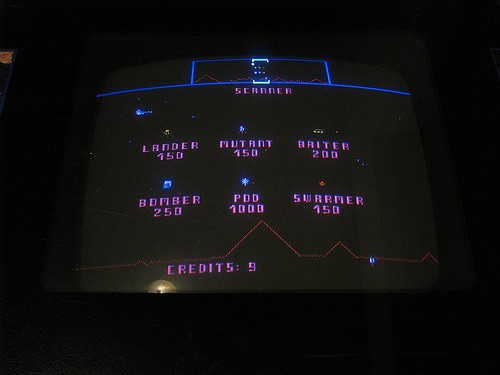The image is a color screenshot of what appears to be a digital screen from an arcade game, set against a completely black background. At the top of the screen, there is a prominent horizontal blue line, with a blue rectangular box centered above it. Below the line, the screen features a list of game-related terms and their corresponding point values, all written in purple text: "Scanner", "Lander 150", "Mutant 150", "Baiter 200", "Bomber 250", "Pod 1000", and "Swarmer 150." Additionally, at the bottom of the screen, the word "Credits" is written followed by a colon and the number "9". Above the word "Credits," there is a stylized pink graph resembling a heartbeat or mountain range. There is also some light reflection visible in the lower-left corner of the screen, indicating it might be a photograph taken in a dark room.